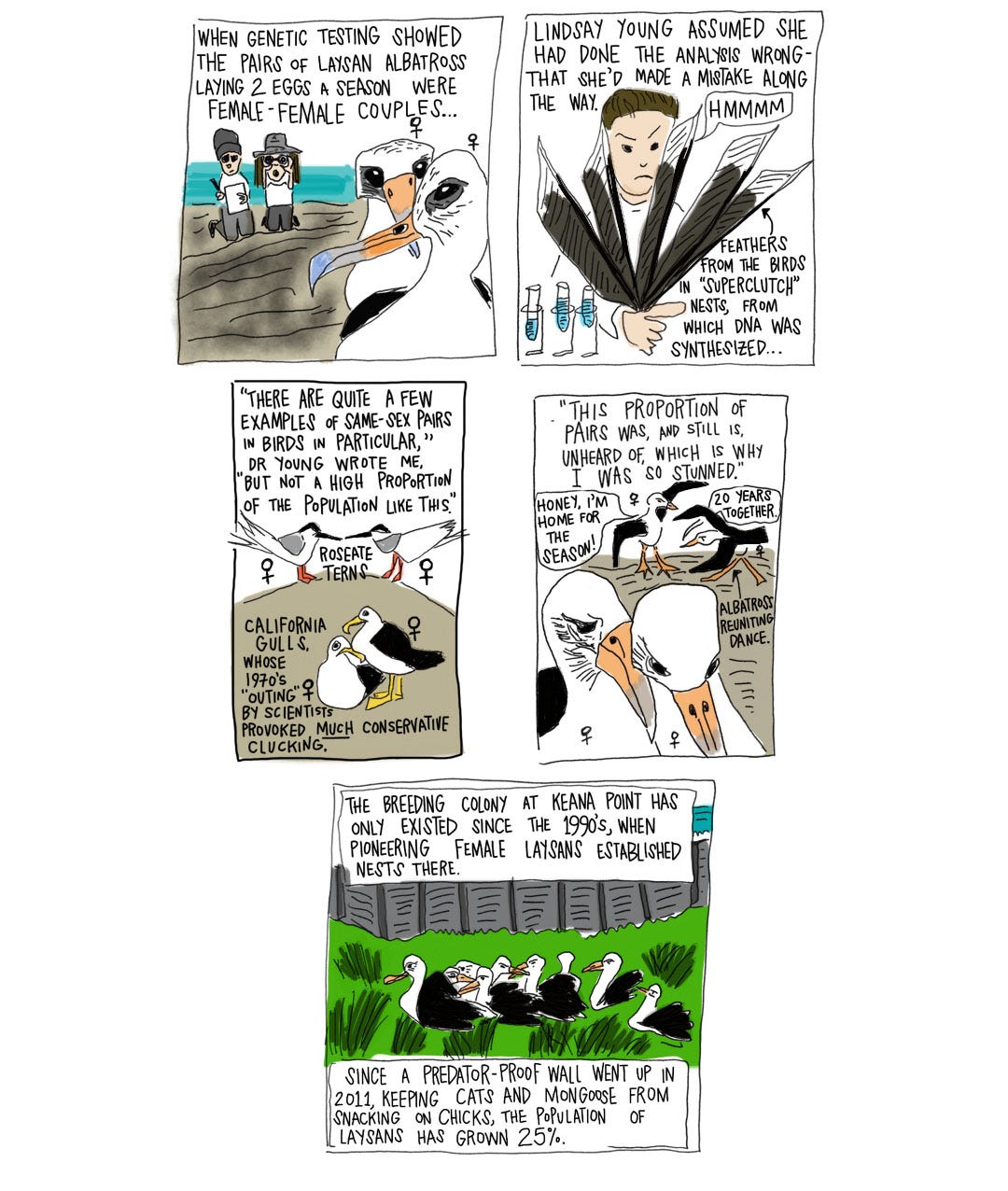This image is a cartoon from either a newspaper or a personal website, featuring a comic strip about two seagulls. The comic, which appears to have an operatic theme, explores the concept of same-sex relationships in nature. One seagull appears to be Cybertron, laying two eggs, while another, a young Asum, does not dance as well. The upcoming character, an MC, seems integral to the storyline. The comic touches on the idea that both female and male same-sex couples can exist in nature, drawing a parallel to human societal norms. Set against the backdrop of the fictional Kenyon Point, a location that closed since the 1990s and saw pioneering women in the leasing business, the comic emphasizes the importance of protecting and ensuring the existence of same-sex couples.